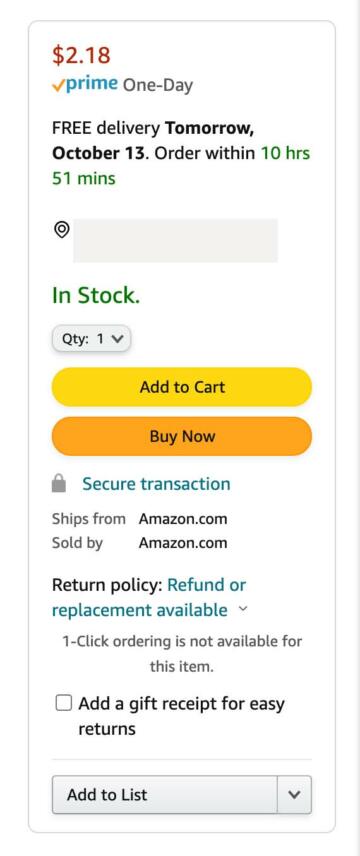This is a detailed view of an Amazon product page interface, focusing on the section where customers can add the item to their cart or buy it immediately.

At the top of the section, there's a white rectangular box outlined in light gray. On the left-hand side, a red dollar sign indicates the price of $2.18. Below this, an orange checkmark is followed by the word "Prime" in blue text, signifying that the item is eligible for Prime delivery. A black text line states "One-Day," referring to the shipping speed, alongside the word "Free" in capital black letters. This line further elaborates that the delivery will be scheduled for tomorrow. 

The next line informs customers that if they place an order within the next "10 hours, 51 minutes" (highlighted in green), they will receive the item the next day, October 13th. Additionally, the term "In Stock" is clearly marked in green.

Further down, there is a small gray rectangle labeled "QTY" (Quantity) with a default number "1" and a downward arrow for adjusting the quantity.

Two clickable ovals are displayed next. The light orange oval says "Add to Cart" in black text, while the darker orange oval says "Buy Now" in white text. 

Beneath these buttons, blue text reads "Secure transaction," followed by black text stating the item "Ships from and sold by Amazon.com." The return policy is highlighted in blue, stating "Refund or replacement available." 

Following this, the interface notes that "One-click ordering is not available for this item." A black-outlined box below offers the option to "Add a gift receipt for easy returns." At the bottom of the section, there is an option to "Add to List."

This detailed breakdown captures the essential elements of the Amazon product purchase interface, ensuring clarity and completeness in the description.